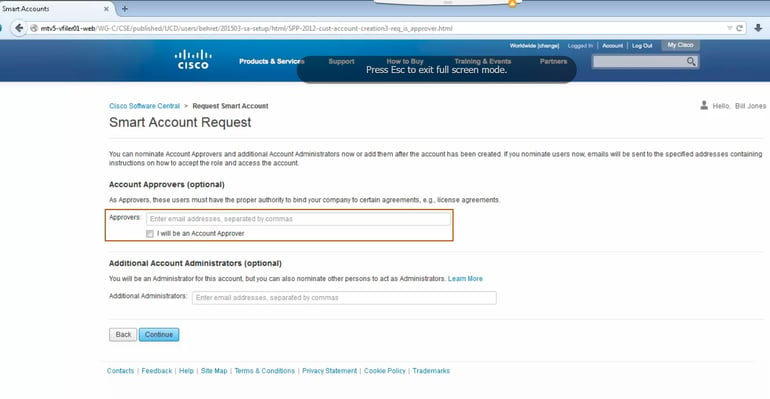"A screenshot of a user interface features a Smart Account request window with an orange box, blue border at the top, and a white background. The window prompts the user to press 'Escape' to exit full-screen mode and contains a search bar, various tabs, and options to go back or cancel. Black text within the window includes 'Profile' and a greeting: 'Hello, Bill Johns.' The header also displays the Cisco logo spelled out as 'C-I-S-C-O' accompanied by an icon of eight white bars."